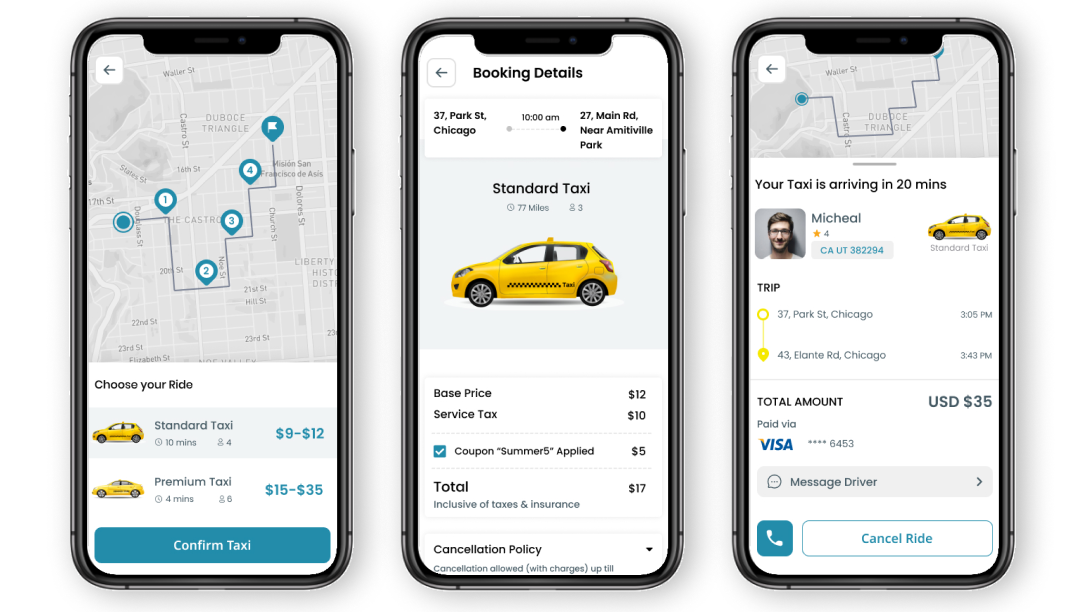This image is composed of three screenshots from a phone, likely an iPhone, given the visible outline of the device. The screenshots depict the process of booking a taxi via a ride-hailing app.

In the first screenshot, a map occupies the upper two-thirds of the screen. Below it, the app displays ride options: "Standard Taxi" highlighted in teal, priced between $9 to $12, and "Premium Taxi" priced between $15 to $35. Users can confirm their selection by clicking a teal "Confirm Taxi" button at the bottom.

The second screenshot shows the "Booking Details" screen, detailing a ride from 37 Park Street, Chicago to 27 Main Street, near Amityville Park. The chosen ride is a standard taxi seating three people. The breakdown of costs includes a base price of $12, a service tax of $10, and a $5 discount from a "SUMMER5" coupon, bringing the total to $17. The screen also shows a cancellation policy at the bottom.

The third screenshot displays a map in the top quarter of the screen, indicating the approaching taxi's location. It shows that the taxi, driven by Michael, is arriving in 20 minutes. Below this, the booking details are reconfirmed, showing a total amount of $17 paid via Visa. Users have the option to message or call the driver, or cancel the ride with buttons at the bottom of the screen.

This detailed sequence illustrates the user's journey from selecting the type of taxi, through booking, to tracking the approaching vehicle.